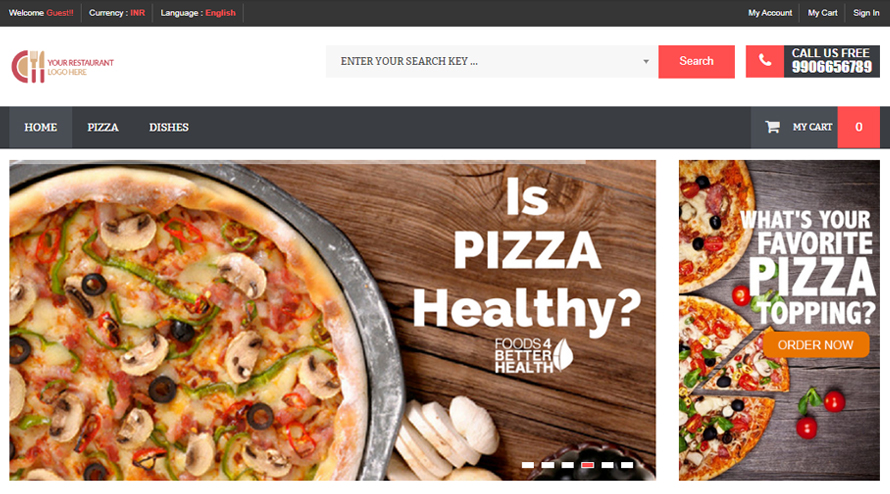Sure, here's the cleaned-up and detailed caption:

---

This cropped screenshot showcases a mock-up of a pizza restaurant's homepage. The layout begins with a thin, black header at the top. On the left side of this header, in white text, it reads "Welcome," followed by "Guest" in red. Adjacent to this is the word "Currency," accompanied by three tiny red letters. Further along, it displays "Language," with "English" highlighted in red. On the far right side of the header, small white letters denote "My Account," "My Cart," and "Sign-In."

Beneath the black header, the background transitions to white. This section contains a half-plate icon flanked by a fork and knife on the left, next to which is a logo placeholder titled "Your Restaurant Logo Here" in red letters. Centrally positioned is a search bar with the placeholder text "Enter Your Search Key," followed by a red search button labeled "Search" in white text. To the right of the search bar is a telephone icon and the text "Call Us Free" in a black box, next to a placeholder phone number.

A thicker black border is situated below this white section. On the left, it lists options such as "Home," "Pizza," and "Dishes." On the right, it shows "My Cart" again, accompanied by a red box with the number "0."

The primary visual element of the mock-up is a large, rectangular image of a pizza in a pan, taking up significant space. To its right is the text, "Is Pizza Healthy? Foods for Better Health." Adjacent to this, a narrow vertical rectangular box displays two pizzas on a table with the caption "What's Your Favorite Pizza Topping?" and an orange "Order Now" button.

---

This description provides a detailed walkthrough of the mock-up's visual and textual elements.